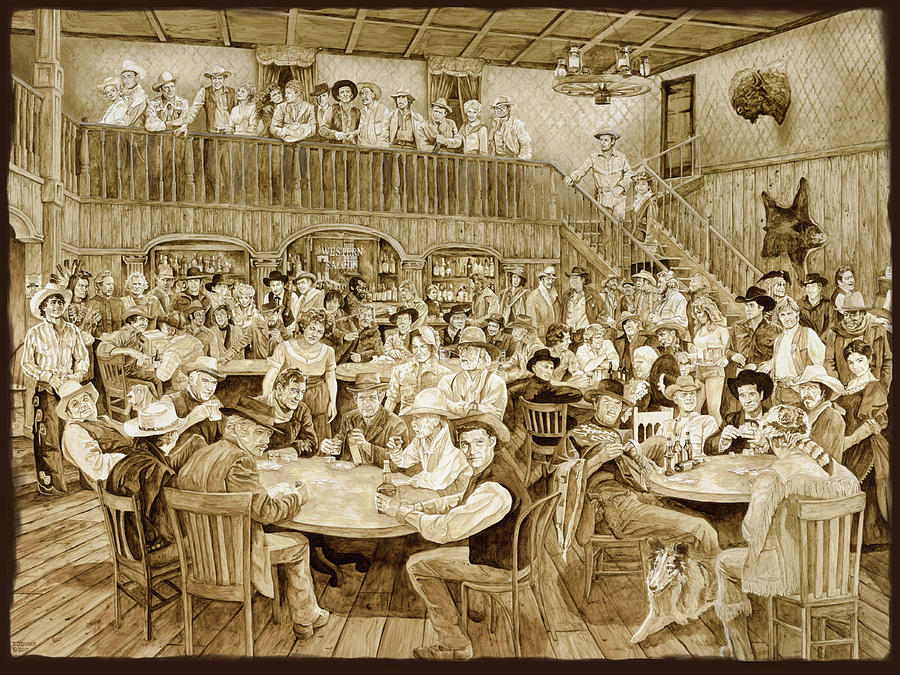In this hand-drawn, sepia-toned illustration of a bustling late 19th to early 20th-century Western saloon, the scene is teeming with life. Inside the mostly brown interior, a bit of white highlights the details, such as the wooden floor and the occupants’ attire. The saloon is crowded with people garbed in cowboy hats, vests, and some even donning coonskin caps. In the foreground, several round tables are filled with patrons—eight individuals occupy the table on the left, while five are at the table on the right, including a man with a coonskin hat in the lower right corner. A collie dog lies on the ground near him. The background reveals a busy bar setup, complete with shelves lined with liquor bottles. Further back, people are either playing poker, engaging in conversations, or standing in clusters near the bar area. The image also features a buffalo head mounted on the wall and a staircase that leads to an upstairs balcony, where more patrons overlook the lively scene below. The overall atmosphere suggests a lively, animated gathering, typical of a Western saloon environment.